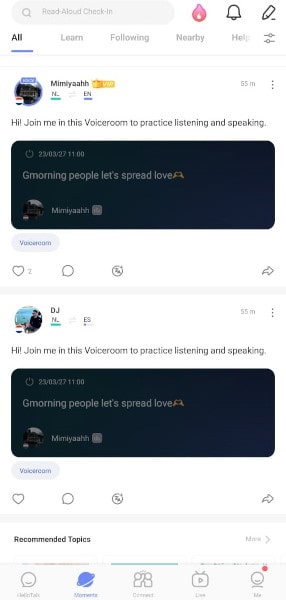The app page features a user interface designed for social interaction and learning. At the top of the page, a search bar labeled "Read Aloud Check-In" is prominently displayed. To the right of the search bar, there is a pink flame icon, followed by a white and black bell icon. Furthest to the right on the top bar is a black and white pencil icon. 

Below the top bar, there are five tabs: "All" (which is currently selected, indicated by a blue line below it), "Learn," "Following," "Nearby," and "Help" (the latter of which is slightly cut off). 

Beneath these tabs, user posts are featured. The first post is by Mimia, identified as a VIP. The text reads, "Hi, join me in this voice room to practice listening and speaking." Below this message, there is an image that says, "Good morning people, let's spread love." This post has two likes, zero comments, and no shares.

The second post is by DJ, and it features identical content: "Hi, join me in this voice room to practice listening and speaking," accompanied by the same image and caption, "Good morning people, let's spread love." This post, however, has no likes, comments, or shares.

Below these posts, a partially visible section titled "Recommended Topics" appears, with a "More" option aligned to the right.